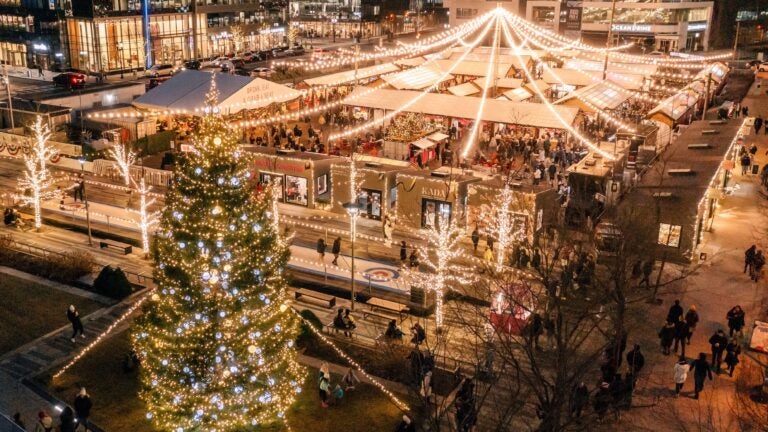The image depicts an enchanting aerial view of Boston's Seaport's Holiday Hub, transformed into a Christmas wonderland. In the foreground stands a colossal Christmas tree, adorned with twinkling white lights and festive ornaments. The guy wires stabilizing the tree are also festively illuminated. Extending behind the tree, the scene captures a tent-like structure formed by strings of Christmas lights cascading from a central point, echoing the design of a circus tent. Beneath this glowing canopy, the bustling hub features numerous market stalls and vendor booths, attracting crowds of people who fill the area with holiday cheer. Surrounding the festive center are bare trees wrapped in lights, benches for visitors, and light-colored buildings that house part of the Christmas market. Further in the distance, the cityscape showcases Boston's illuminated office buildings, adding an urban backdrop to the holiday display. The entire scene is vibrant and lively, perfectly embodying the festive spirit of the season.